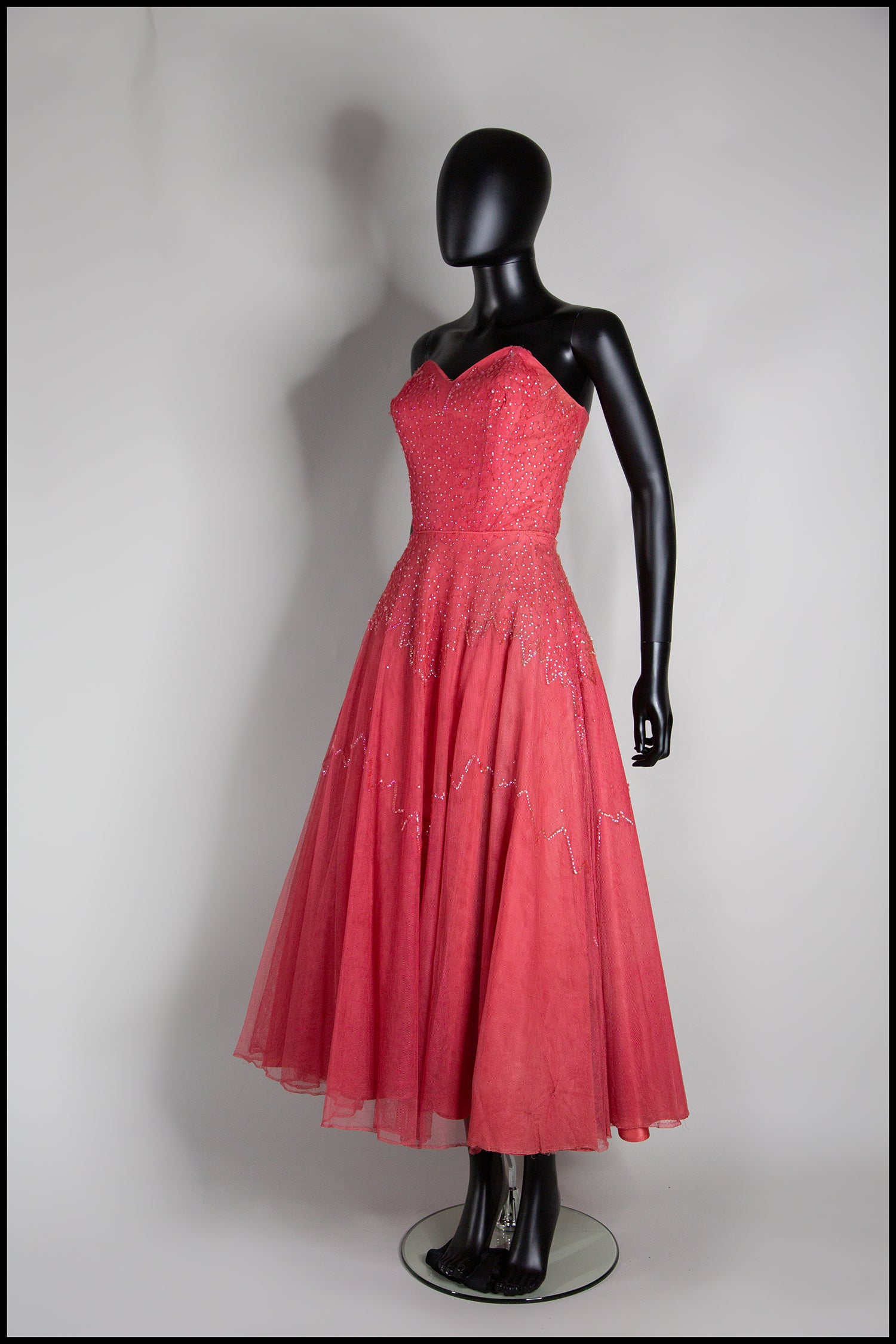The photograph features a highly stylized black mannequin with a sleek, featureless face and an elongated, slender form, positioned against a light gray background. The mannequin casts a dark gray shadow against this backdrop, enhancing the depth of the image. The figure is adorned in a stunning, strapless red dress that extends nearly to its ankles. The dress is exquisitely detailed, featuring a form-fitting beaded bodice that accentuates the mannequin's chest, and flares out into a flirtatious, layered skirt with a sheer top layer. The left arm of the mannequin is posed back, giving it an elegant, poised stance. Its feet, designed for high-heeled shoes though currently bare, rest on a clear, transparent disc, completing the mannequin's refined presentation.